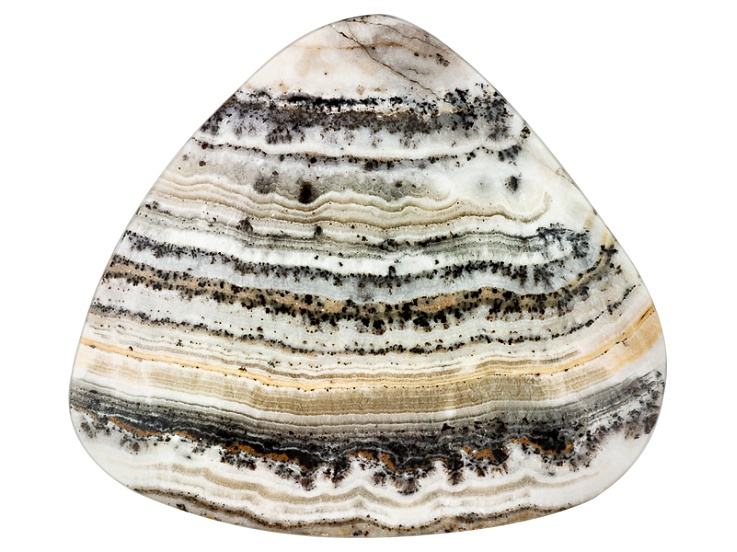The image is a highly detailed, close-up photograph of a naturally layered object, likely a rock or shell, set against a completely white background. The object is shaped like a softened triangle or a wide pear and features a multitude of curved, horizontal striations. These layers, which span a range of colors from white to cream, tan, brown, black, and even a hint of very light purplish near the top, suggest it is either a polished rock or a cross-section of one. The surface appears shiny, emphasizing its detailed and varied hues. The photograph’s close-up perspective highlights over a dozen distinct layers within the object, though the lack of any scale reference in the background makes it difficult to discern its actual size. There is also a small crack visible near the top, adding to its natural intricacy.